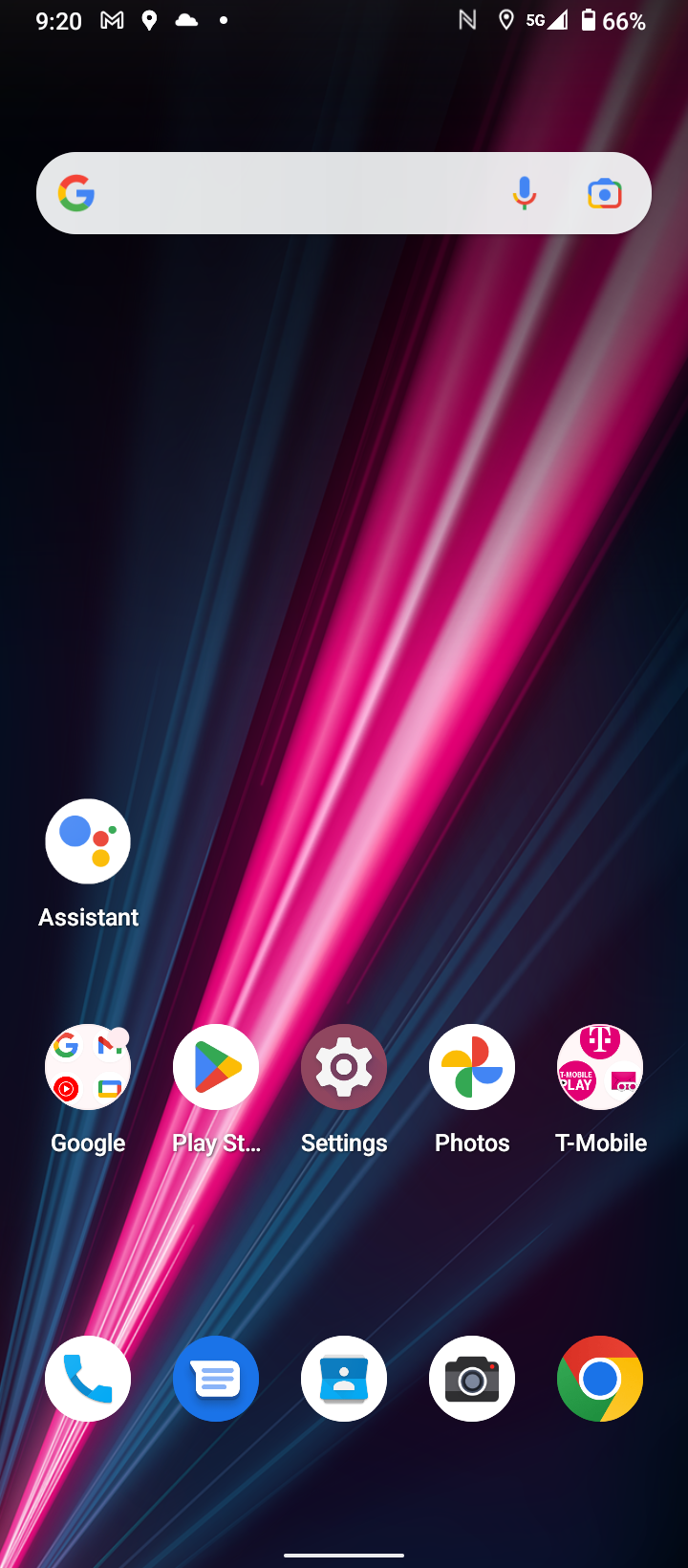The image showcases a sleek, modern smartphone with a distinctive almost-phone-like appearance. The screen is active, displaying a simplistic yet visually appealing home screen, characterized by a cohesive color scheme. Most prominently, the screen features a circular arrangement of widgets and icons, deviating from the conventional square icons. Notable icons include the familiar Google apps—Camera, Phone, and Messages—indicative of its Android operating system. At the top of the screen, indicators for notifications, battery level, signal strength, and time are neatly aligned, providing essential information at a glance. Dominated by Google's ecosystem, the display includes recognizable Google Search and Google app icons in their signature green and red hues, reinforcing the device's identity as a Google phone.